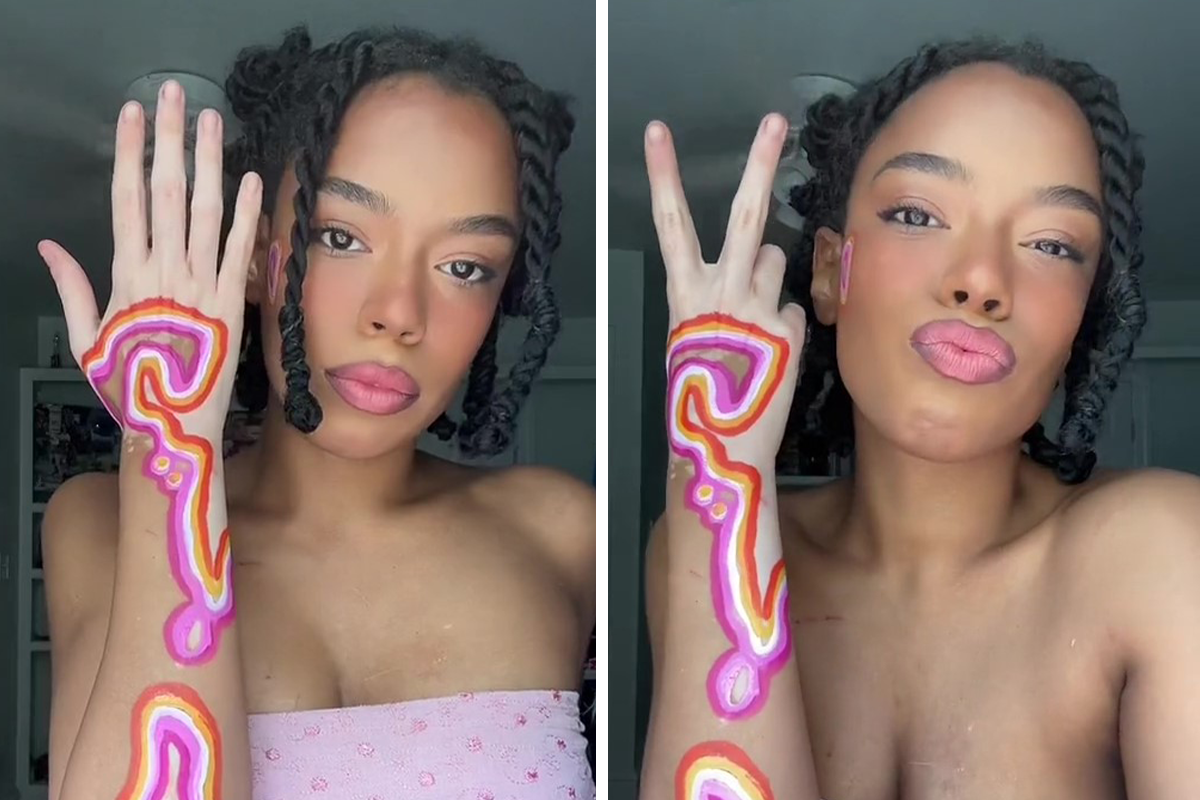In the side-by-side images, a brown-skinned girl with braided hair is captured taking selfies. She has vibrant pink lips outlined in brown and wears a pink tube top. The left image shows her staring directly at the camera, with her left arm raised and fingers outstretched, displaying intricate red, orange, white, and pink paint drawings on her hand and forearm. Her hand is notably lighter than the rest of her body, suggesting a skin condition. In the right image, she makes a kissy face at the camera and flashes a peace sign. Additionally, a heart painted in matching colors decorates her cheek, and her tube top seems to have fallen out of frame. Her makeup is striking, with prominent blush and bright pink magenta lipstick enhancing her features.